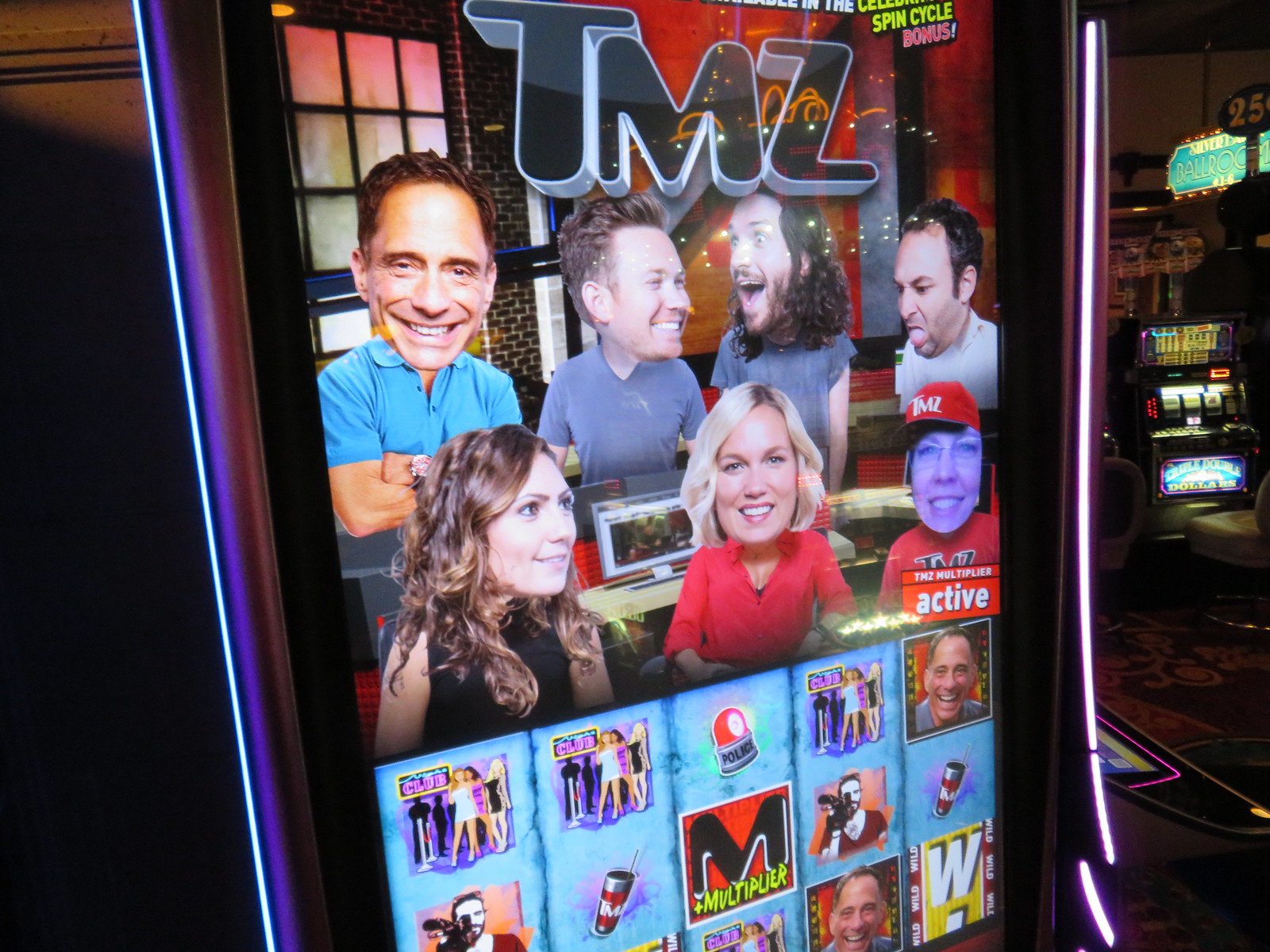This detailed image captures a TMZ-themed slot machine located in a casino. At the top of the machine, "TMZ" is prominently displayed in big black letters. Below, the screen showcases seven people from the TMZ show arranged in rows—four men on top and three women beneath them. The woman positioned in the middle of the bottom row has short blonde hair and wears a red shirt. These individuals display varied facial expressions, adding a dynamic element to the scene. The slot machine features five vertical columns with five rows, packed with various symbols typical of such games. 

Above the slot reels, the words "TMZ Multiplier Active" are highlighted in red. The machine's sides are adorned with neon lights, transitioning from purple on the right to blue on the left, adding a visually appealing, inviting aura. The surrounding casino floor, seen to the right, is decorated with funky designs. Adjacent to the TMZ machine, another slot machine displays "Double Dollars," and a yellow "Ballroom" sign is visible in the upper right corner of the image, enhancing the casino atmosphere.